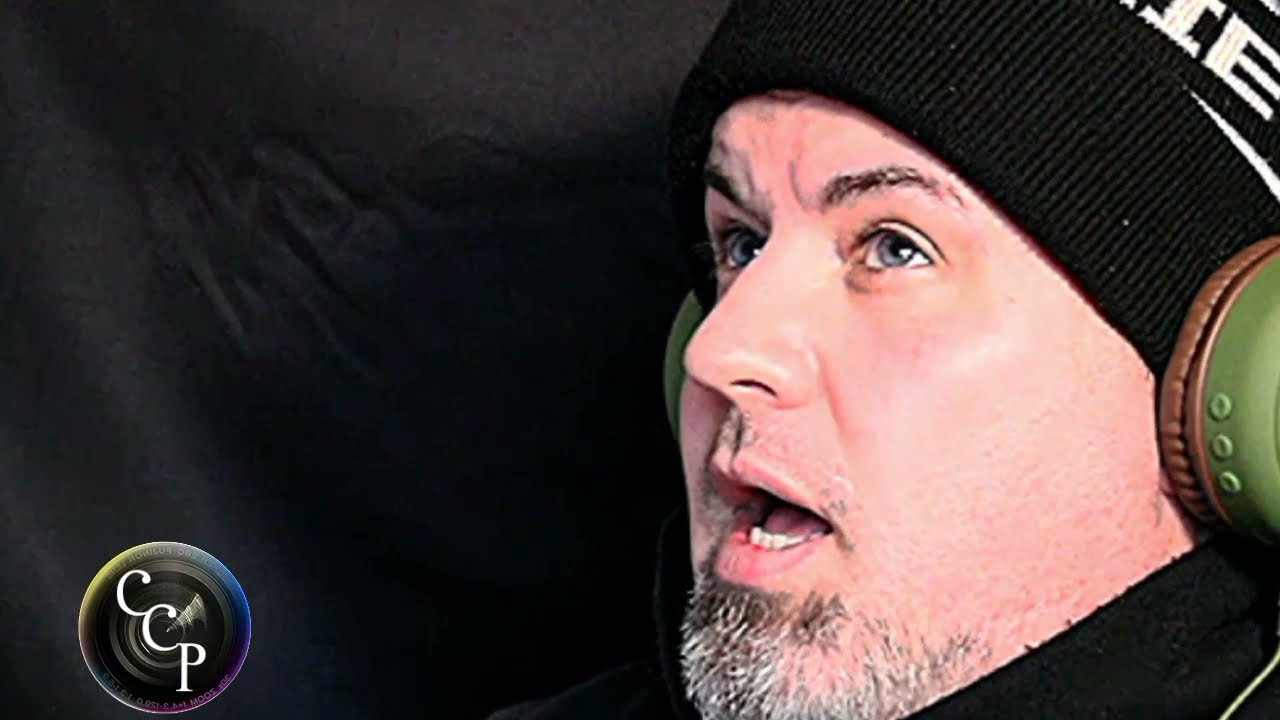This is a close-up, horizontally-oriented color photograph featuring a man's face against a predominantly black background. The man is positioned on the right side of the image, with his head and collar visible from his chin to his forehead. He has fair skin and a scruffy gray and black goatee with splotches of whiskers but no full mustache. His mouth is open as if he is speaking or singing, and his blue eyes are looking upwards. He wears a black beanie cap adorned with white letters, partially showing "IE," and green headphones bordered in brown. He is also dressed in a black jacket, though only the collar is visible. To the left side of the image, in the bottom left corner, there is a circular, speaker-like shape with white letters "C.C.P" diagonally arranged from the upper left to the lower right. This circle, along with the predominantly black background, adds a stark contrast to the detailed depiction of the man's expressive face.